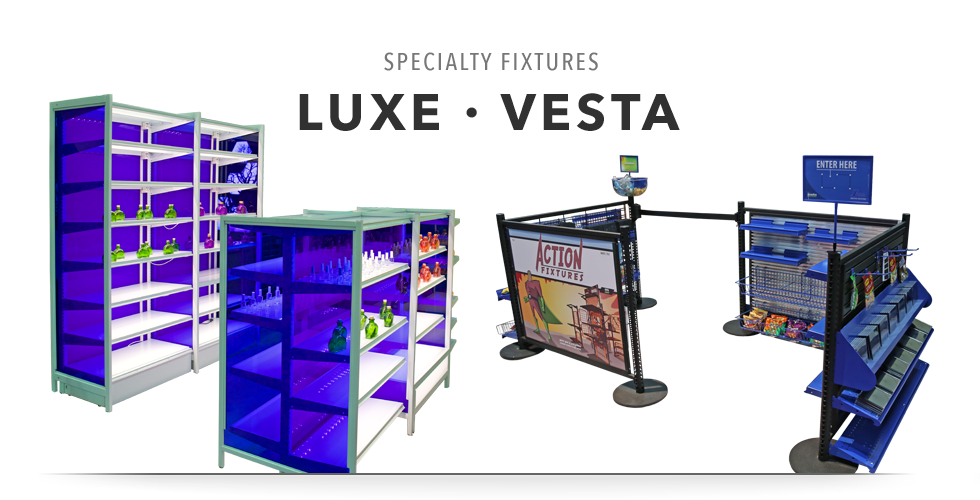The image showcases a detailed diagram of various retail display fixtures under the brand Specialty Fixtures by Luxe Vesta. At the top, there's a grey title reading "Specialty Fixtures," followed by the bold, dark, and prominent title "Luxe Vesta." The display features a range of shelving units and display cases, each meticulously detailed. On the left side, there are multiple shelving units, each with blue transparent glass exteriors and white shelves, containing green and purple objects as examples. These shelves include both tall single-sided shelving units and more complex double-sided aisle units designed to be placed in store aisles. Towards the right, there are modules meant for queue lines, including barricades and hanging shelves intended for last-minute purchase items such as candy bars. Additional elements include room dividers with pamphlet holders and small signboards, suggesting their use in a convention or retail setting to direct customer flow and display additional merchandise.